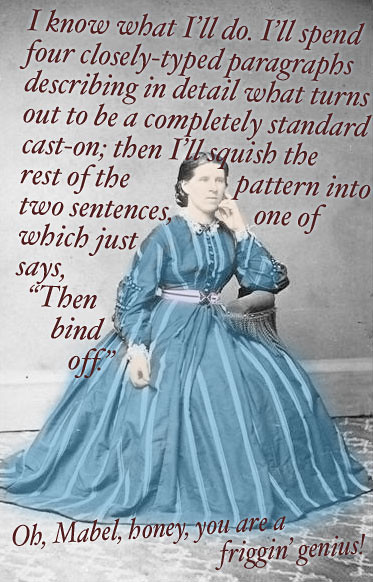The image is a close-up of a museum display featuring a colored photograph of a woman named Mabel. In the photo, an old black-and-white image has been colorized to show Mabel in a blue dress with light blue stripes. She is seated, posing with her head resting thoughtfully on her closed fist, showcasing her short hair. Above and behind her, the wall text humorously reads, "I know what I'll do. I'll spend four closely typed paragraphs describing in detail what turns out to be a completely standard cast-on. Then I'll squish the rest of the pattern into two sentences, one of which just says, then bind off. Oh, Mabel, honey, you are a friggin' genius!" The specific context or date of the photograph isn't provided, nor is the title of the display clarified, leaving the viewer to ponder the witty commentary on knitting instructions.